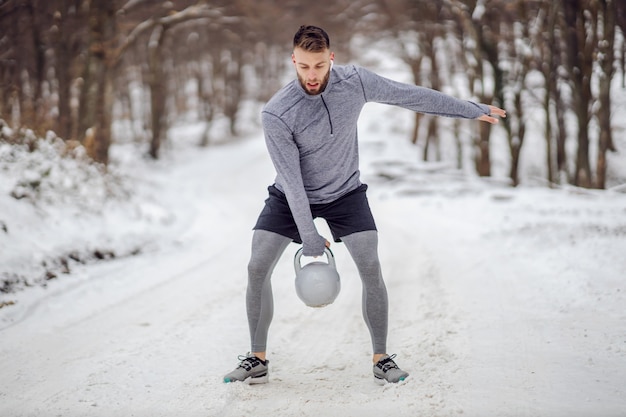The photograph captures a man amidst a snowy landscape, possibly during a workout or exercise photoshoot. The man, of Caucasian descent with short brown hair, a beard, and a white Bluetooth earpiece in his ear, stands in the center of the image. He is wearing a long-sleeved gray zip-up jacket that extends over his palms, black or dark gray shorts over gray leggings, and gray sneakers with black accents. His outfit, suitable for cold weather, suggests it's a chilly environment.

He is positioned on a snow-covered road, with barren trees featuring brown trunks and no leaves visible in the background. The midday light reflects off the snow, adding to the wintry atmosphere. The man is slightly bent at the knees and waist, looking down as he struggles to balance while holding a heavy gray kettlebell in his right hand. His left arm is extended straight out to the side, contributing to a dynamic and intense pose that emphasizes the physical effort he is exerting.